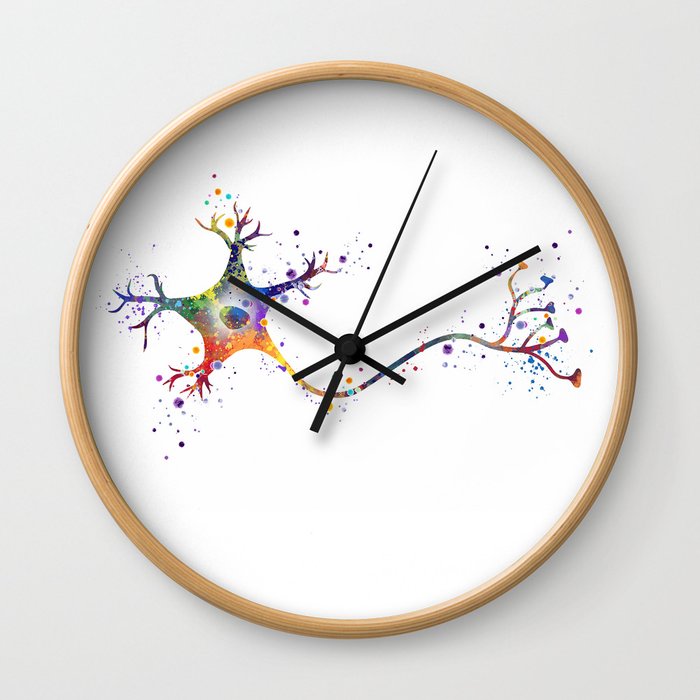The image features a square composition with a soft, light gray or off-white background suggesting a wall. Centrally hung on this backdrop is a large, circular clock framed by a narrow wooden border that resembles bamboo in color. The clock is distinctive for its minimalist design, lacking any numerical indicators. Instead, it features three thin black hands—hour, minute, and second—that point in different directions from a shared circular center. 

The clock's face is primarily white, serving as the canvas for an intriguing, colorful graphic resembling a starfish or a biological organelle. This vibrant image spans the middle section of the clock, with the top and bottom portions remaining blank. The graphic art showcases a blend of rainbow colors, including green, blue, purple, red, and yellow, and features a central thick line with branching elements like pods or tree limbs that extend on both sides. The organism-like design has five tips resembling a star and exhibits fine branching details at the ends. This unique and abstract artwork adds an eye-catching focal point to the clean, modern aesthetic of the clock.